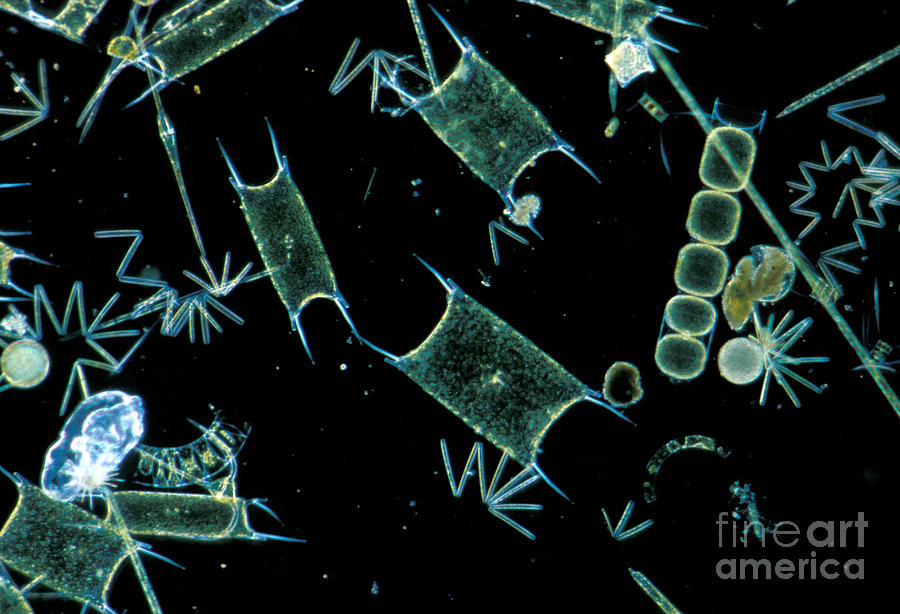The image, marked with a "Fine Art America" watermark in the bottom right corner, showcases a highly detailed, digitally created piece that mimics the appearance of various microorganisms or cells viewed through a microscope. Featuring a horizontal rectangular format, the composition displays a broad array of shapes and sizes scattered across a stark black background. The color palette includes vivid blues, greens, yellows, and subtle hues of beige, white, and gray. Central to the image are the largest organisms, displaying unique and unusual forms such as rectangular shapes with green or blue protrusions resembling horns, and peculiar structures akin to conjoined 'W's. Surrounding these primary forms are numerous other elements including pill-like clusters, spider-like shapes with round bodies and extending legs, as well as oval and zigzagged figures. Additionally, small dots are speckled throughout the image, enhancing the microscopic effect. The artistic style emphasizes abstract and surreal interpretations of what could be cellular forms, arranged at diverse, often diagonal angles, creating a visually intriguing tableau.